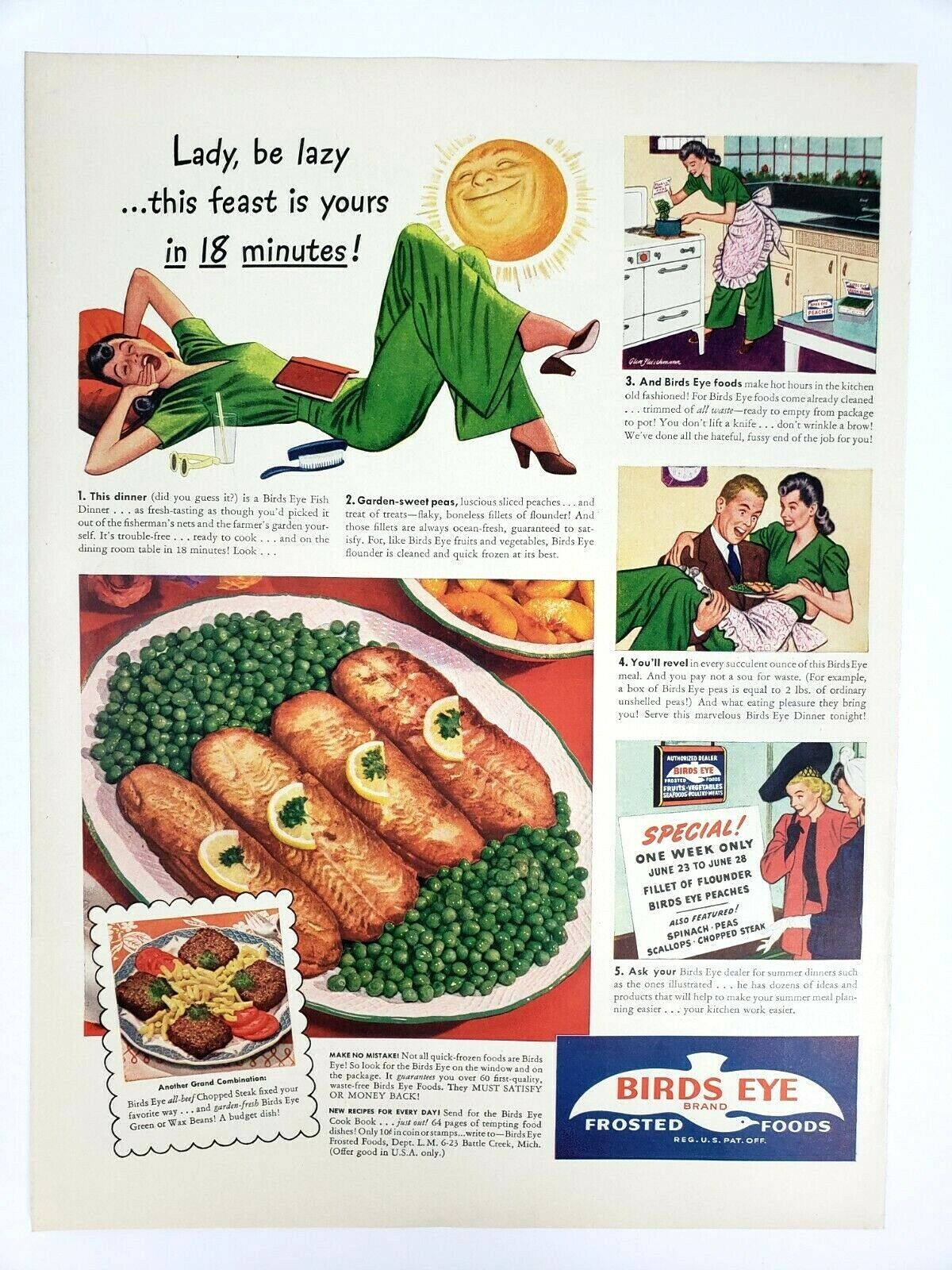This image depicts a vintage advertisement, likely from the 1950s, with the headline "Lady, be lazy. This feast is yours in 18 minutes" written in black font at the very top. The central illustration portrays a woman in a green dress reclining with her head on a pillow, a book resting on her stomach, an empty glass nearby, along with a pair of sunglasses and a brush. Above her, a smiling sun adds a whimsical touch. Text is scattered throughout the image, though much of it is small and difficult to read.

Below the relaxed woman is an illustration of a plated dish, potentially featuring fish or salmon fillets, garnished with peas on either side. To the top right, a separate section includes another depiction of the woman, now in an apron, pouring a bag of peas into a pot in a kitchen setting. Adjacent to this, we see the same woman joyfully holding the completed dish while embraced by a man, presumably her husband. This sequence suggests the ease of meal preparation promoted by the ad. At the bottom right, an additional panel features two women examining a sign that reads in red, "Special," followed by black text detailing a limited-time offer: "One week only, June 23rd to June 28th, fillet of flounder, Bird's Eye, peaches."